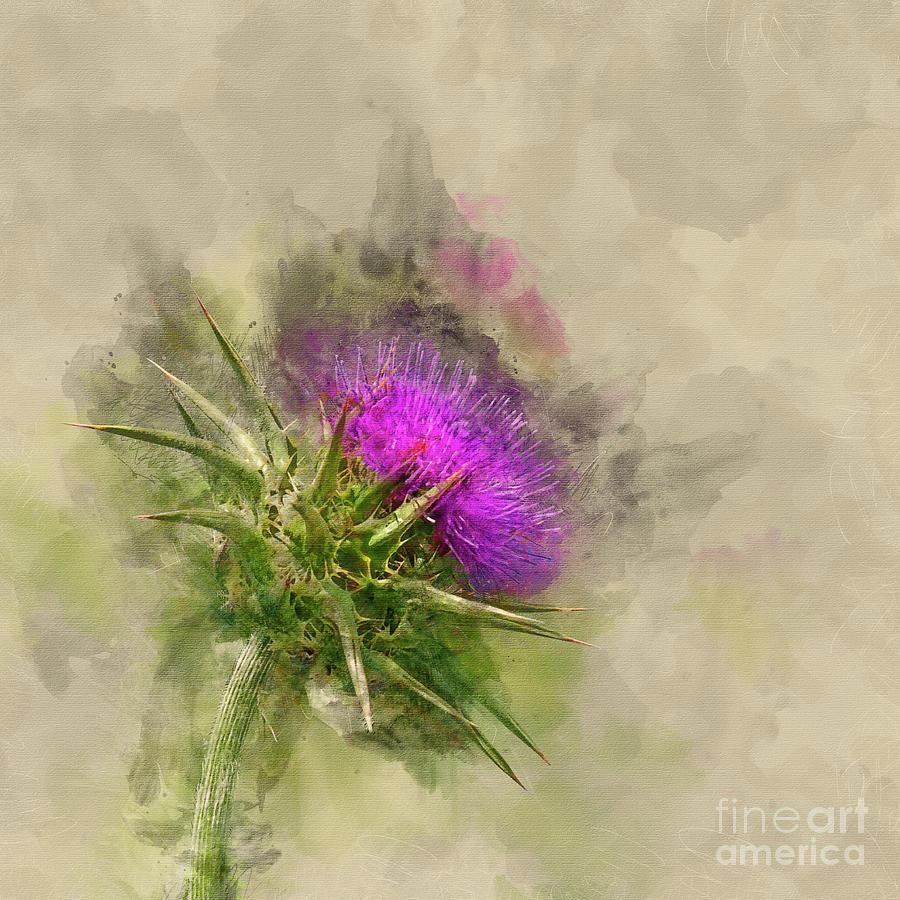The image depicts a painting featured on Fine Art America, indicated by the subtle watermark in the bottom right corner. The background is a blend of abstract, mottled patterns with hues of light green, brown, and gray, creating a textured and layered effect. At the center of the composition is a detailed and vibrant thistle plant. The thistle's centerpiece is a rich purple flower, surrounded by green, spiky leaves and thorns. The stem extends downwards to the lower left, contributing to the artwork's dynamic nature. The background's abstract elements include smudges and stains, adding depth and a cloud-like quality to the overall scene. An artist's signature, beginning with the letter 'A', is faintly visible in the upper right corner of the painting. This intricate artwork contrasts its finely detailed focal point with the abstract, watercolor-like surroundings, offering a complex visual experience.